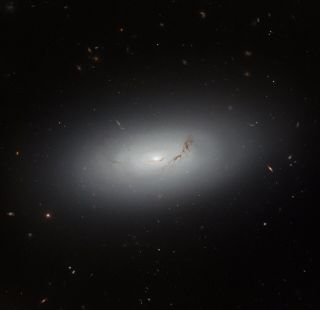The image appears to be a deep space photograph, possibly taken by a powerful telescope or artistically rendered. Dominating the composition is a central feature that could either be a white planet or a galaxy, characterized by a distinct white glow. This central object is surrounded by a swirling disk or rings of dust, with a faded, oval-shaped aura spreading outward. Just to the right of this bright focal point, there's a noticeable brownish discoloration, possibly an anomaly. The backdrop is predominantly black, speckled with numerous small white dots, some larger than others, likely representing distant stars or planets. The striking contrast between the central luminous body and the dark, sparsely dotted expanse enhances the sense of cosmic vastness and isolation.